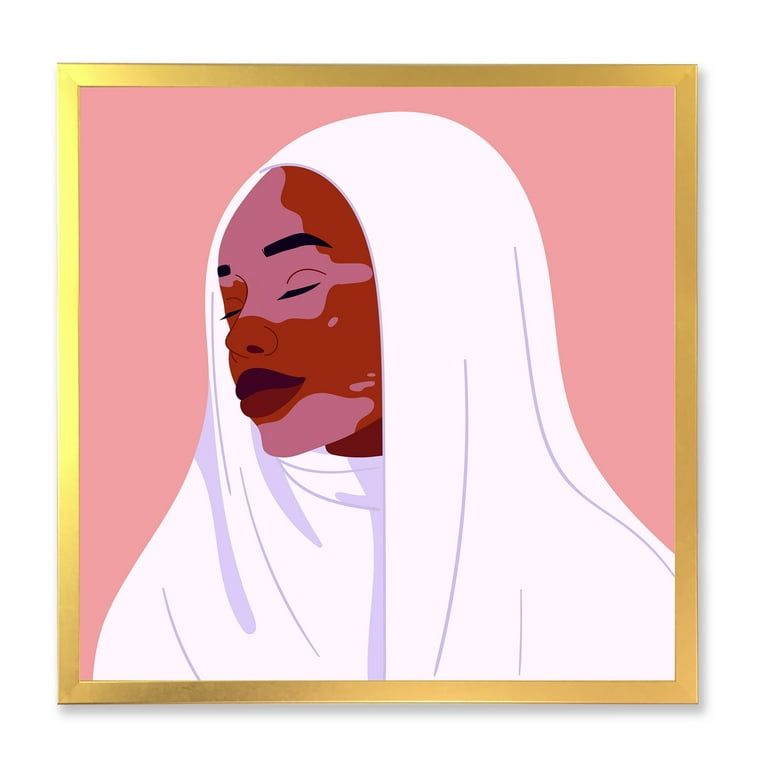This image is a detailed painting of an African-American woman, emphasizing her serene and introspective demeanor with her eyes closed and her head tilted to her right, our left. Enclosed in a gold frame, the background of the image is a soft pink-peach color, creating a warm and gentle contrast to her dark, rich skin tones. 

Her skin shows a unique blend of dark browns and lighter patches, which resemble vitiligo, with areas that almost match the pink of the background. Her facial features include dark, thick eyebrows and long dark eyelashes framing her closed eyes, and full lips painted in a striking dark red. She wears a flowing white veil or scarf, which could be interpreted as a hijab, gracefully draped over her head and shoulders, concealing her hair and extending down to cover much of her upper body. There are subtle, intricate details on the fabric of the veil, adding to the ethereal quality of her portrayal.